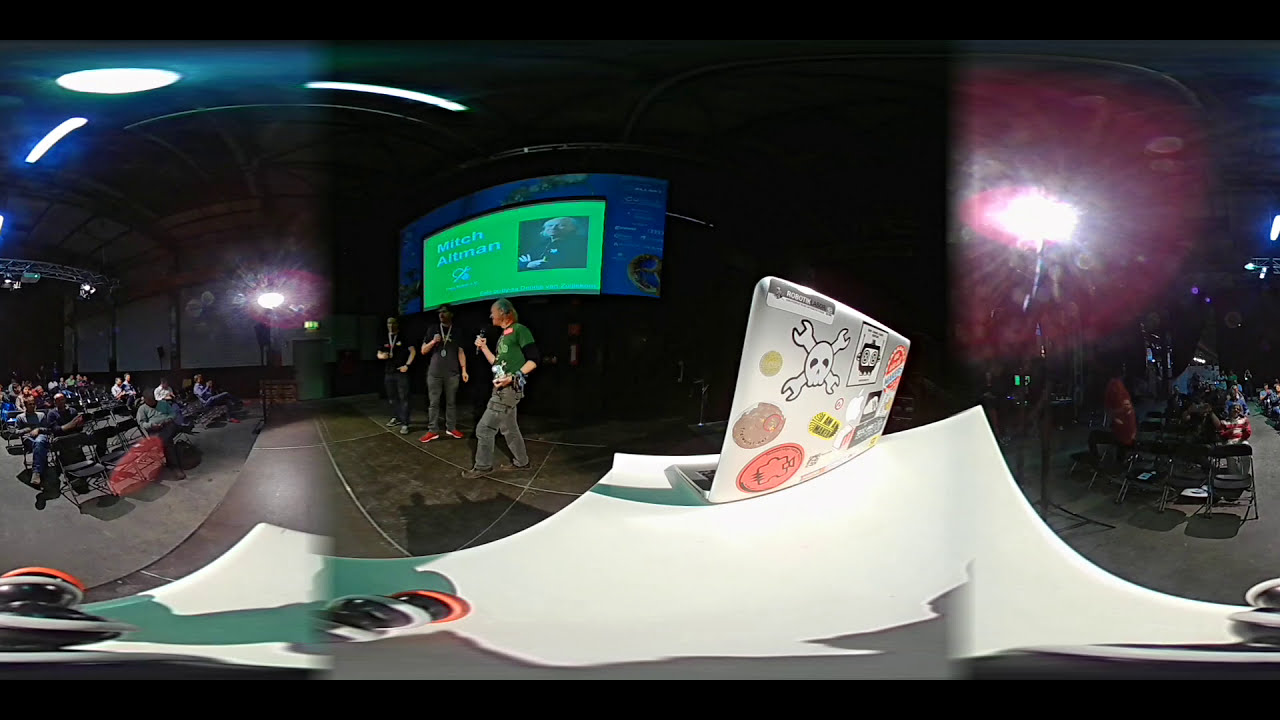The image captures a casual, indoor musical presentation or small concert in progress, taking place on a black stage. There are three individuals on the stage, each holding microphones. The one on the right is wearing green-gray trousers, while the two on the left are in blank shirts. Above them hangs a large green screen with the text "Mitch Altman" in white, alongside an indistinct photograph of a man with crossed arms. Due to the 360-degree lens distortion, the audience appears split across two separate sections, with attendees seated in fold-out chairs on either side of the stage. Below the stage, a white table or desk holds an open silver laptop adorned with various stickers, including a skull and crossbones with spanners. The room, dimly lit except for light sources flanking the stage, suggests a casual and informal atmosphere, possibly a fun post-work activity or casual concert.